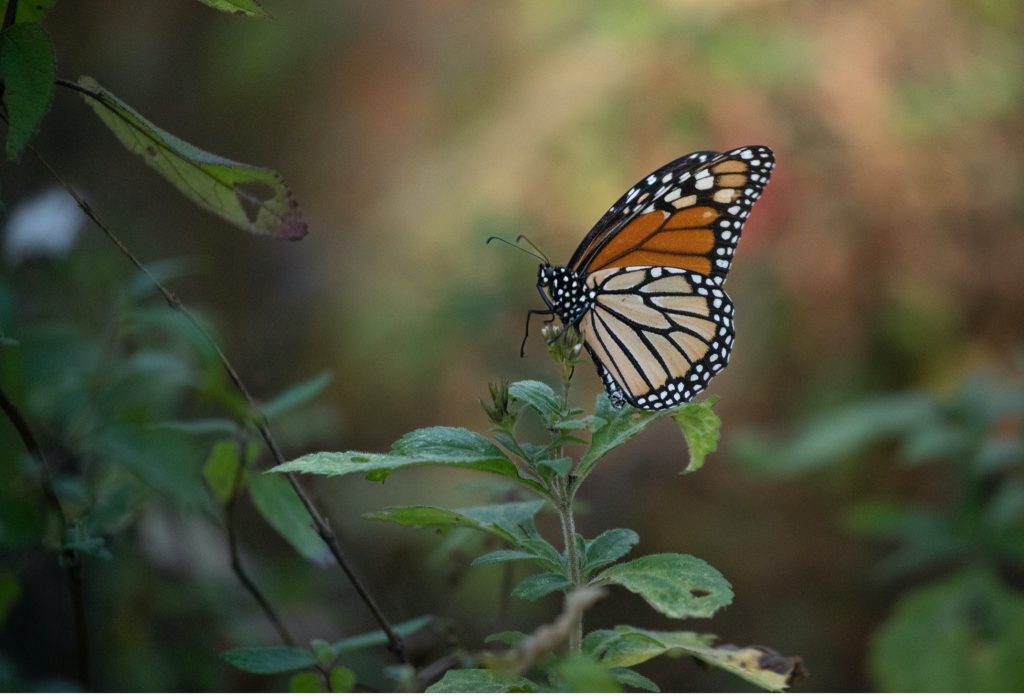The image captures a stunning, clear wildlife photograph of a classic monarch butterfly, viewed from its left side with its wings elegantly displayed. The monarch, identifiable by its striking orange wings accented with black veins and white spots along the edges, rests atop an unidentified green plant. The plant appears lush, with many leaves clearly visible in the foreground, along with some similar plants nearby, suggesting a garden setting. Though the exact plant type is not confirmed, it could possibly be milkweed, known to attract monarchs.

The butterfly's wings are positioned almost upright, partially open so both the outer and inner sections are visible. The wings exhibit a gradient of orange shades, darker in the upper sections and lighter in the lower. The butterfly's black body is adorned with white spots, and one leg juts out to the left at a right angle, while its long antennae extend gracefully from its head. 

The photograph, captured in landscape orientation, features a backdrop that is beautifully blurred, enhancing the focus on the butterfly. Despite the shadowed lighting, the subject remains in sharp, vivid detail, making this image not only picturesque but also suitable for identification purposes in field guides or textbooks. In the background, hints of green foliage and a faint pinkish-red tinge add a touch of color to the natural, garden-like setting.